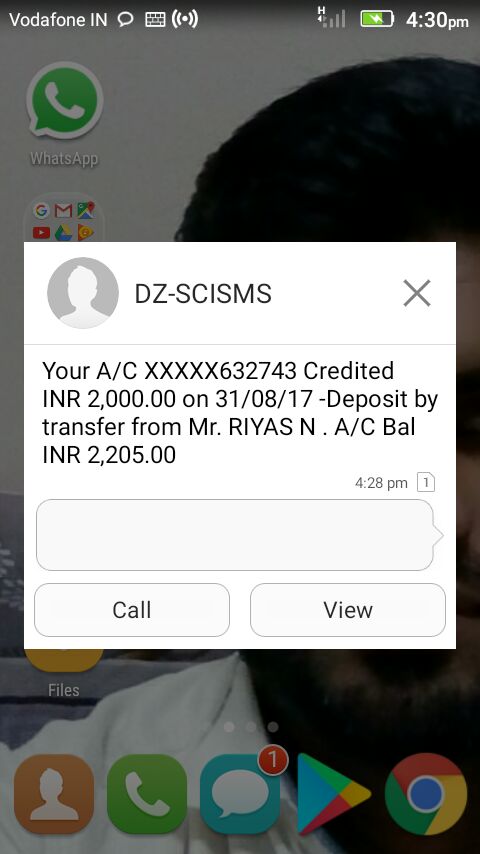The image is a detailed screenshot of a phone's home screen displaying a bank notification. The phone shows Vodafone IN in the upper left corner, while the upper right corner indicates a Wi-Fi logo, a battery icon around three-fourths full, and the time at 4:30 PM. The background features a partially obscured photo of a man with black hair, a beard, and brown skin, wearing doctor's scrubs.

In the center, a prominent white dialog box occupies the screen, overlaying the background image. At the top of this box, the name "DZ-SCISMS" is displayed near an icon of a face. The notification reads, "Your A/C XXXXX632743 credited INR 2000 on 31/08/17," indicating a deposit by transfer from Mr. Rios N. The account balance listed is INR 2205. Below this, the time is noted as 4:28 PM. The dialog box features buttons for "Call" and "View," which are available for further actions.

At the bottom of the home screen, various app icons are visible, including Google Chrome, Google Play, a messaging app, a phone app, and contacts, along with multiple clickable emojis.